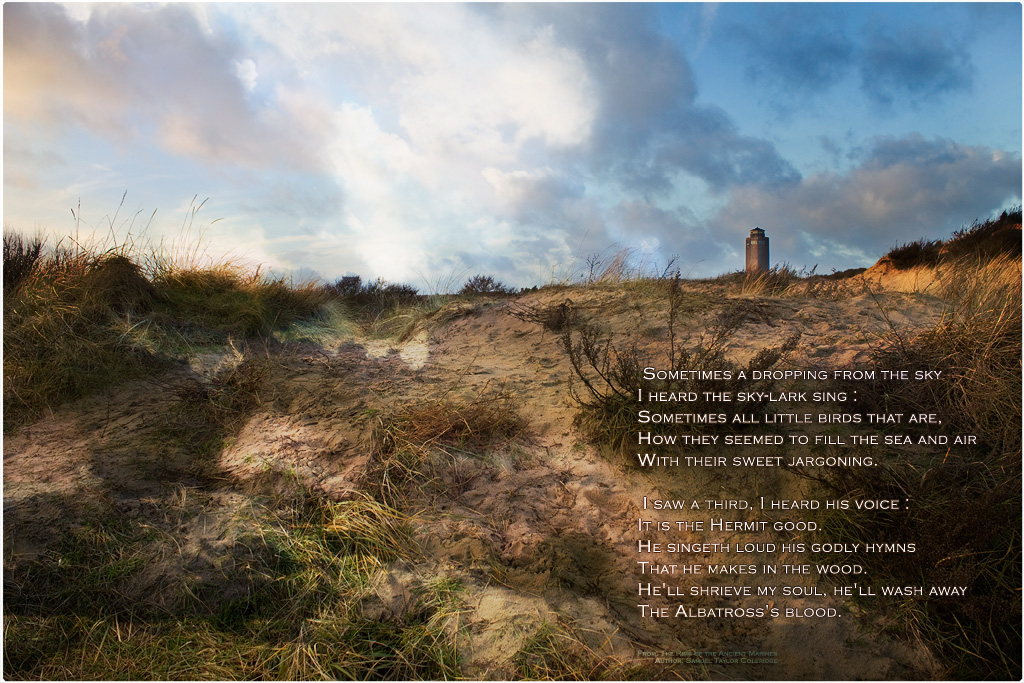The image resembles an inspirational poster capturing a dramatic scene. At the base of a gently sloping hill, a figure stands, gazing skyward. The landscape is a mix of sandy dunes interspersed with patches of long green grass and sparse vegetation, including brown weeds, tumbleweeds, and old bushes. Amidst the greenery, a distinct, dead patch can be observed. In the distant horizon, a solitary, tall, rectangular tower, brown or possibly black with a small dome, stands upright. The sky overhead is a tapestry of dense clouds with varying hues—from brilliant white at the center to amber-tinged edges, set against a deep blue backdrop, giving the impression of a setting sun. In the lower right corner of the image, there is an evocative string of white text which reads: "Sometimes a dropping from the sky, I heard the skylark sing. Sometimes all little birds that are, how they seem to fill the sea and air with their sweet jargoning. I saw a third, I heard his voice. It is the hermit good. He singeth loud his godly hymns that he makes in the wood. He'll shrieve my soul. He'll wash away the albatross's blood."